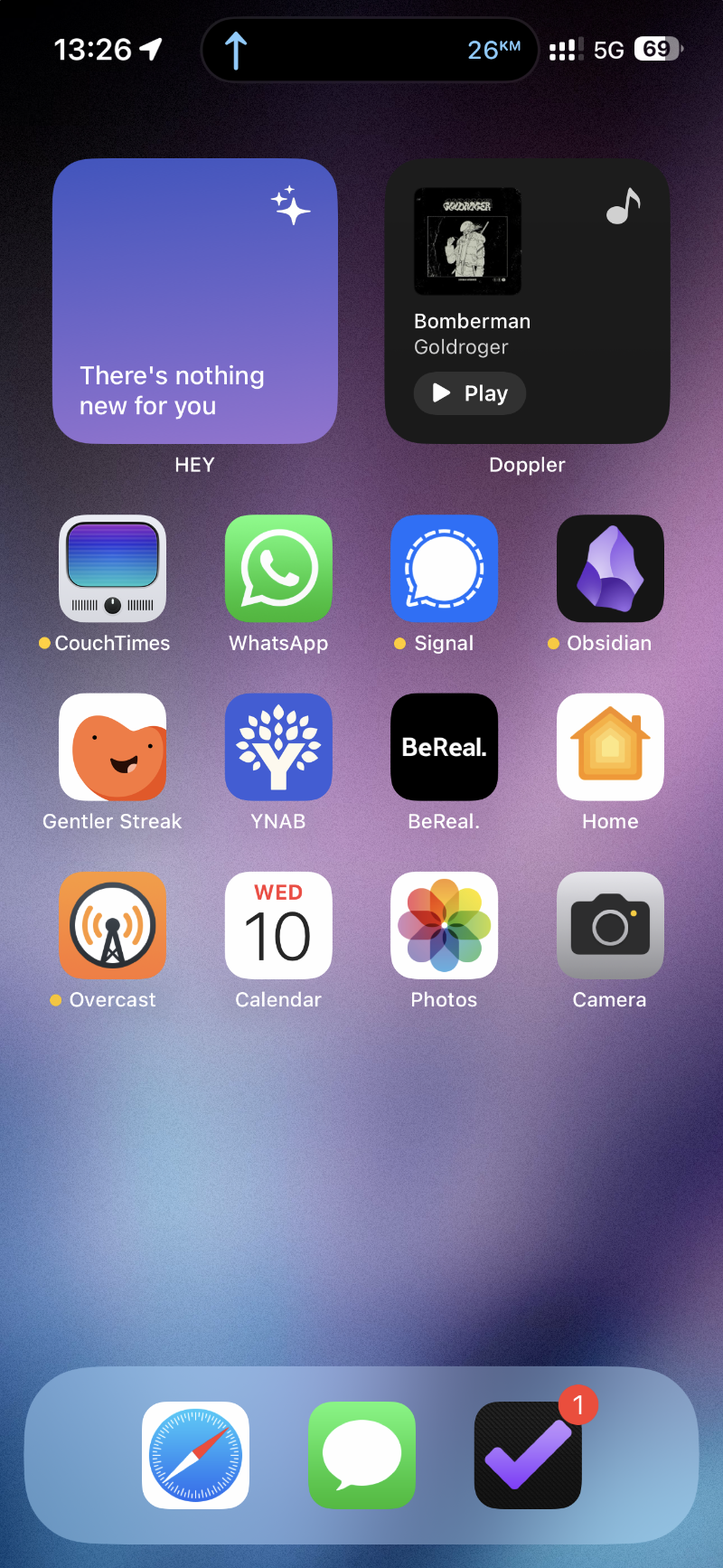The image depicts a smartphone screen displaying a vibrant gradient background and various app icons. The background transitions smoothly from black at the top to lighter purples and blues at the bottom, adorned with swirling patterns throughout.

In the upper-left corner, the time is displayed in white digits, "13:26," accompanied by a small white arrow. Next to it, there’s a search bar with a blue arrow pointing vertically, and the word "kilometers" written in blue. The reception bars, divided in the middle and colored white, are followed by the "5G" label. The battery icon, showing 69% charge, is also present, with the left side in white and the right side in gray.

Below this, a lavender square with three white stars in the top-right corner contains the text, "There's nothing new for you," and below that, "HEY." Adjacent to this square is a dark gray, almost black, square featuring an indistinguishable album cover of a person against a black background. Above the person is unreadable text, with "Bomberman" written below in white, followed by "Gold Roger" in white. A light gray play button, with a white play arrow, is positioned at the bottom. A white musical eighth note is in the top-right corner of this square.

Below this section, there are multiple app icons arranged in a 4x3 grid. The first row features:

1. A gray TV screen icon with a rainbow gradient (purple, blue, light blue) and "Couch Times" written below with a yellow dot beside it.
2. A pinkish-orange bagel or heart icon with black dots and a smiley face, set on a white background, titled "Gempler Street."
3. An orange square showing a gray transmission tower with orange curved lines, titled "Overcast" with a yellow dot next to it.

The second row contains:

1. A green square with a white speech bubble icon, titled "WhatsApp."
2. A blue square with a stylized tree, titled "YNAB."
3. A white square with the red abbreviation "WED" (for Wednesday), the number "10" in black, and "Calendar" in white.

The third row includes:

1. A blue square with a white speech bubble outlined in a dotted line, titled "Signal" with a yellow dot beside it.
2. A black square labeled "BeReal" with "BeReal" written inside.
3. A white square featuring a color palette arranged like a flower, with semi-transparent ovals in red, orange, yellow, green, light blue, dark blue, purple, and purplish-red colors, titled "Photos."

The final row contains:

1. A black square with a stylized violet rock, titled "Obsidian" with a yellow dot beside it.
2. A white square displaying an orange idealized house, titled "Home."
3. A gray square with a black camera icon, titled "Camera."

At the very bottom, a row of three square icons appears:

1. A white square with a blue and red compass icon.
2. A green square with a white speech bubble icon.
3. A black square with a violet checkmark and a red notification circle with the number "1" in white.

The meticulously detailed layout showcases a rich visual experience with a variety of functional elements tailored for smartphone users.